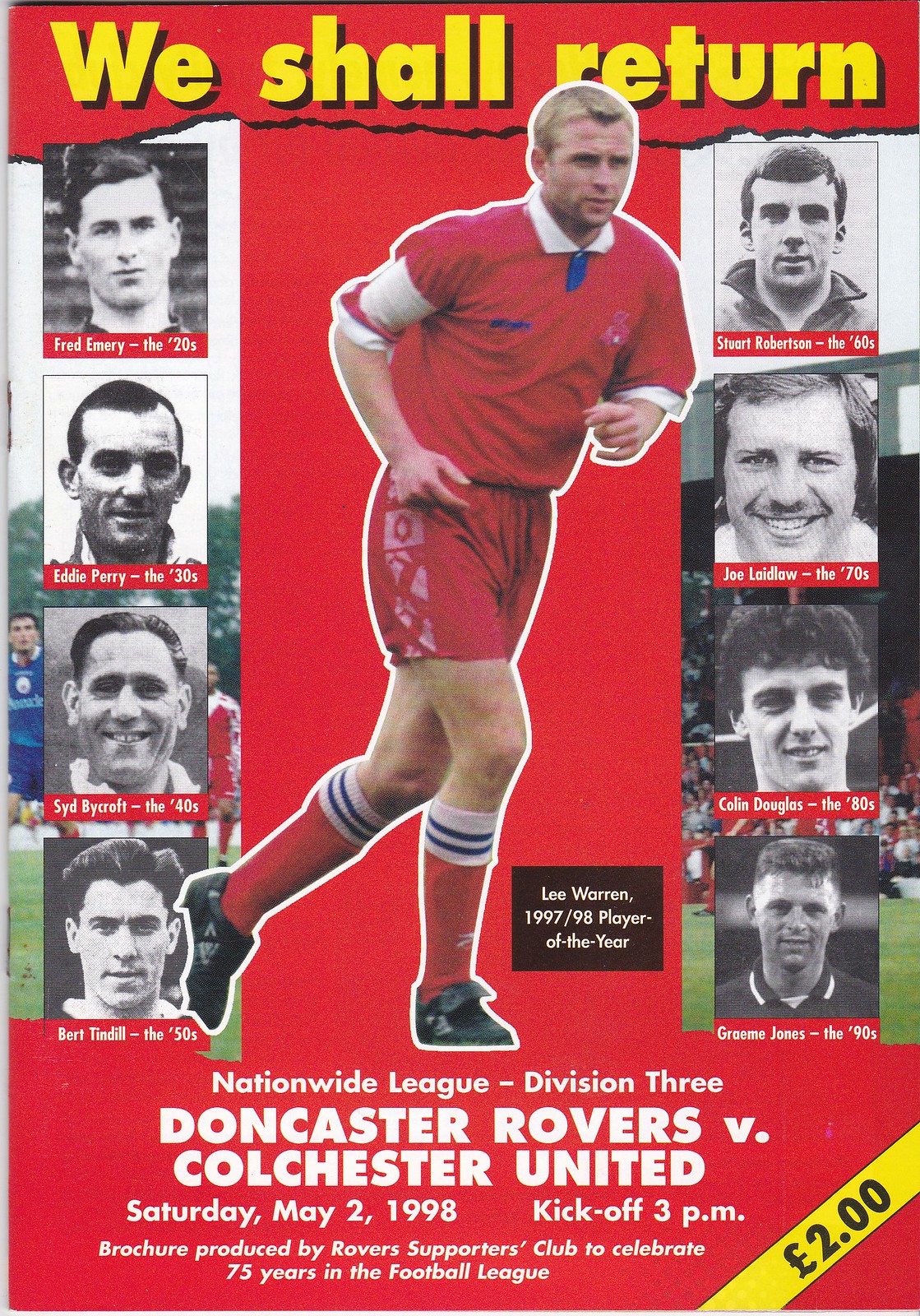The image is of a red brochure for the Doncaster Rovers football club, featuring the title "We Shall Return" in bold yellow font at the top. The central image showcases a player in mid-game action, wearing a red jersey, red shorts, red socks, and black shoes—identified as Lee Warren, the 1997-1998 Player of the Year. Surrounding him are up-close, black-and-white headshots of notable players from different decades, with four on each side. These players include Fred Emery (1920s), Eddie Perry (1930s), Sid Bycroft (1940s), Bert Tindall (1950s), Stuart Robertson (1960s), Joe Laidlaw (1970s), Colin Douglas (1980s), and Graham Jones (1990s). Below these elements is the event information: Nationwide League Division III match, Doncaster Rovers vs. Colchester United, taking place on Saturday, May 2, 1998, with a kickoff at 3 p.m. The brochure is produced by the Rovers Supporters Club to celebrate 75 years in the Football League.